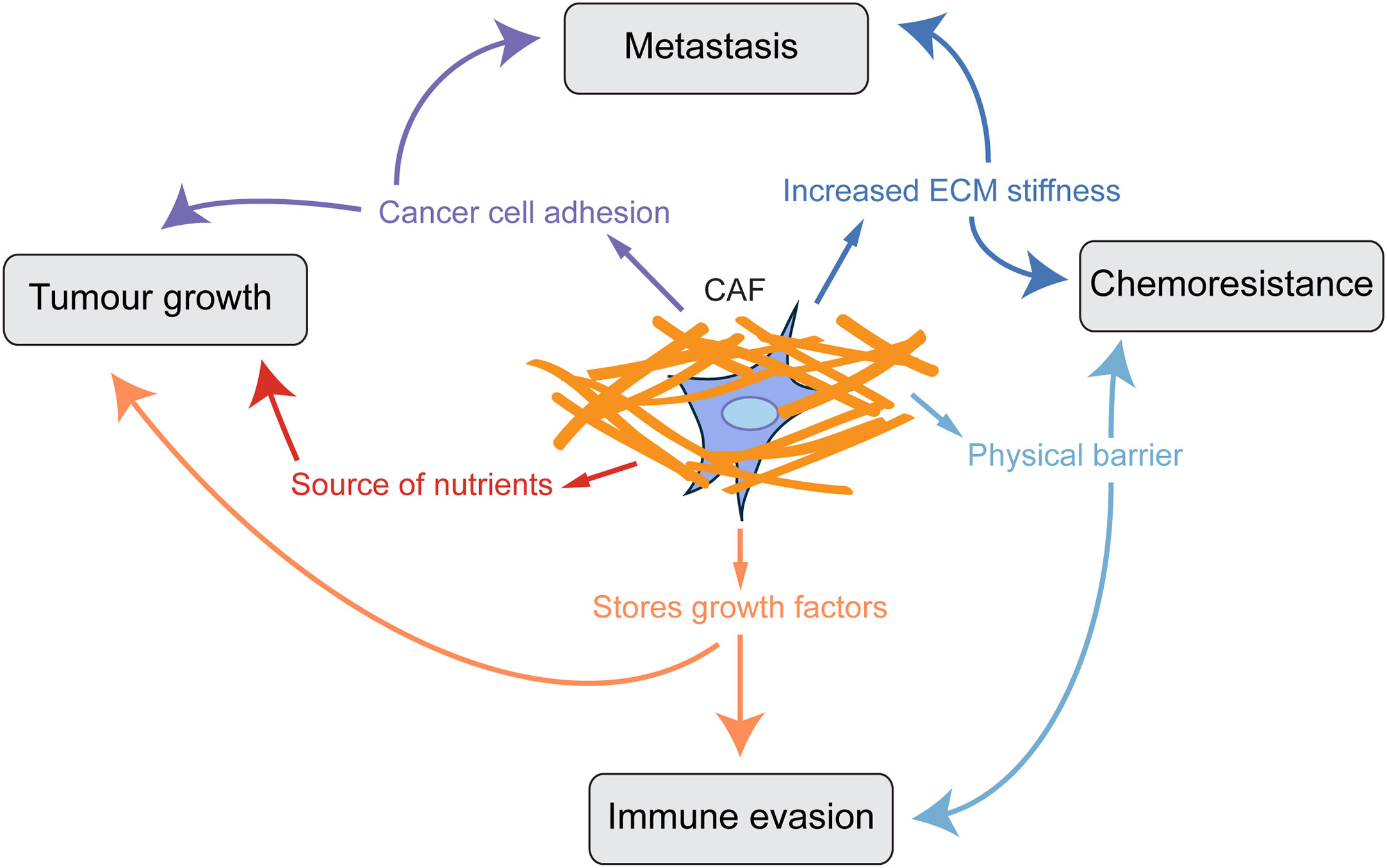The diagram illustrates the complex interactions involved in cancer cell adhesion and metastasis on a white background. At the top, there's a black-outlined box labeled "Metastasis" in black lettering, receiving inputs from two sources: a purple arrow labeled "Cancer Cell Adhesion" and a blue arrow labeled "Increased ECM Stiffness."

In the center of the diagram is a star-like CAF (Cancer-Associated Fibroblast) structure, characterized by an aqua blue circle surrounded by blue and orange crisscrossing lines. This central CAF structure directs arrows both horizontally and vertically affecting various outcomes. From the CAF, an orange arrow labeled "Stores Growth Factors" splits into two: one arrow points downward towards a gray box labeled "Immune Evasion" and another points left towards a box labeled "Tumor Growth." Additionally, a red arrow labeled "Source of Nutrients" also leads from the CAF directly to the "Tumor Growth" box.

Further interactions are detailed as follows: the "Cancer Cell Adhesion" box sends purple arrows towards both "Tumor Growth" on the left and "Metastasis" on the right. The box labeled "Increased ECM Stiffness" connects to "Metastasis" via a blue arrow and to "Chemoresistance" also via a blue arrow. Additionally, from the CAF, a blue arrow labeled "Physical Barrier" points upward towards "Chemoresistance" and another arrow extends to "Immune Evasion."

Overall, the diagram depicts a network of cancer processes, emphasizing the central role of CAF in mediating multiple pathways influencing tumor growth, chemoresistance, and metastasis, interconnected through a series of colored arrows and labeled boxes.